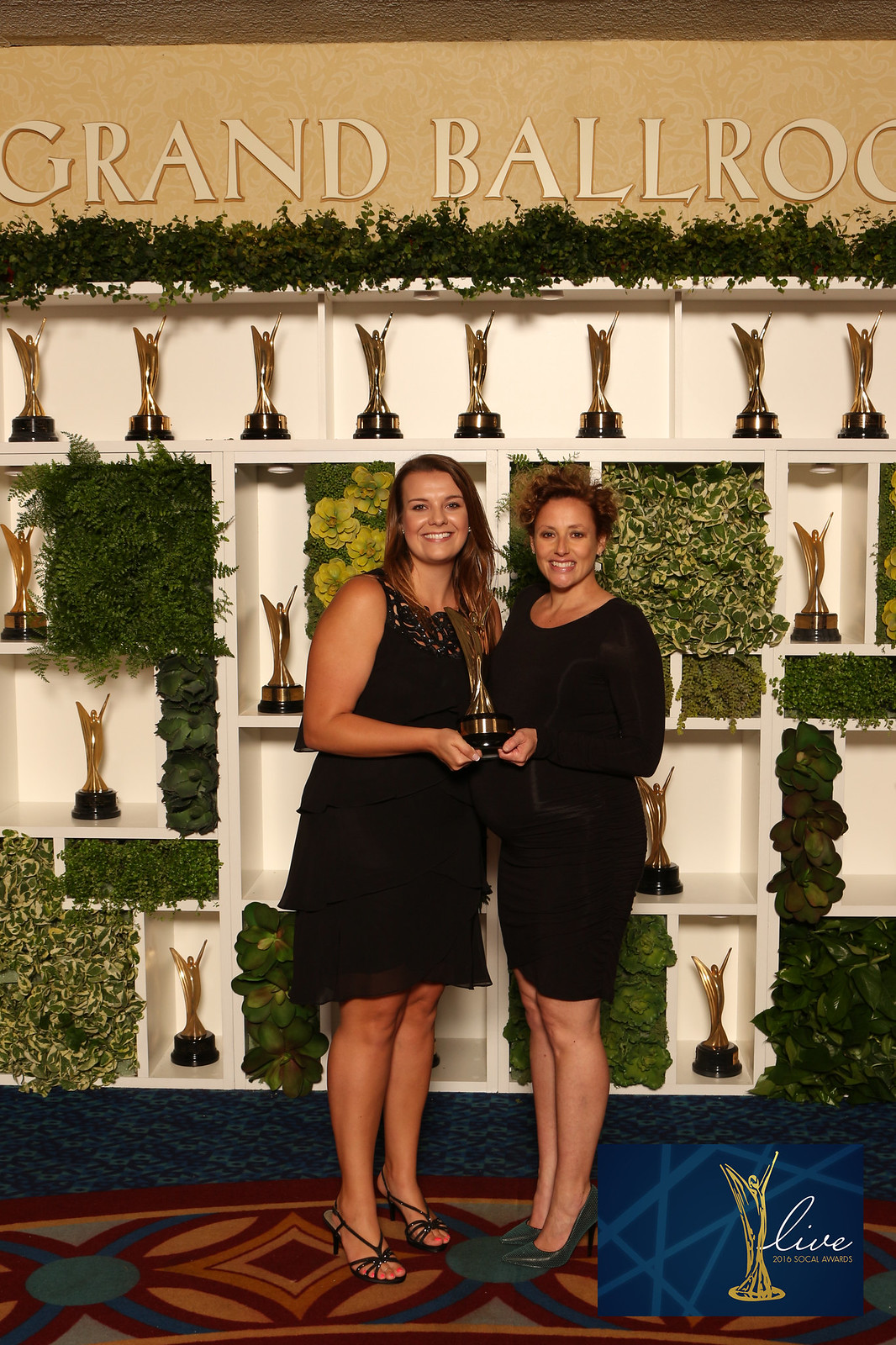In the photograph taken indoors, two brunettes of European descent are standing shoulder-to-shoulder, smiling and looking directly at the camera in front of a white shelving unit filled with gold trophies and potted plants. The women are both wearing black knee-length dresses and high-heeled shoes—one with black open-toed heels showing pink toenails, and the other with gray closed-toe pumps. They are holding a large, gold trophy together, each with one hand supporting it underneath. The trophy features a figure with outstretched arms that resemble wings, and it has a black base. 

Behind them, the top shelf of the unit displays nine identical trophies, and the shelves below house a mix of trophies and plants. Above them, a dark brown banner with whitish print reads "Grand Ballroom." The carpet is patterned with blue, burgundy, yellow, and beige geometric designs, and additional blue carpet and foliage feature behind the shelving unit. In the lower right-hand corner of the image, there is a blue square with a gold statue and white print that says "LIVE." In gold print, it states "2016 Social Awards."